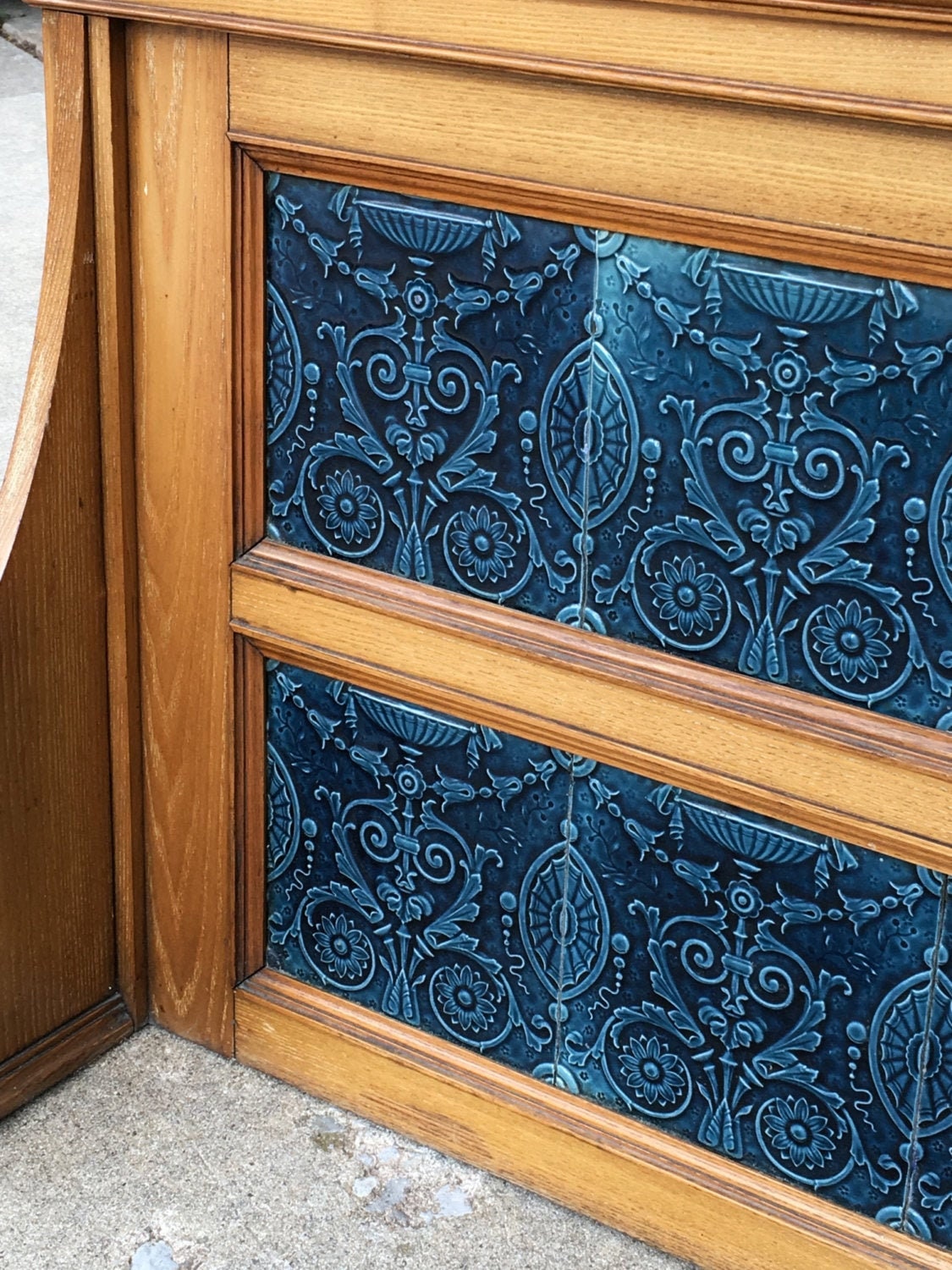This image features a cropped view of a two-drawer dresser made of solid brown-stained oak wood, set against a brown tile floor. The dresser showcases ornate, dark metal engravings with lighter silver accents in the center of each drawer. The metalwork is intricate, featuring circular and oval scrolls, a vase-like design, and rows of flowers. The detailed engravings resemble a chalice or birdbath with additional elements such as hearts, tulips, and vines. This unique and elaborate design, despite the partial view only showing the middle and bottom drawers, highlights the piece's sophisticated craftsmanship.